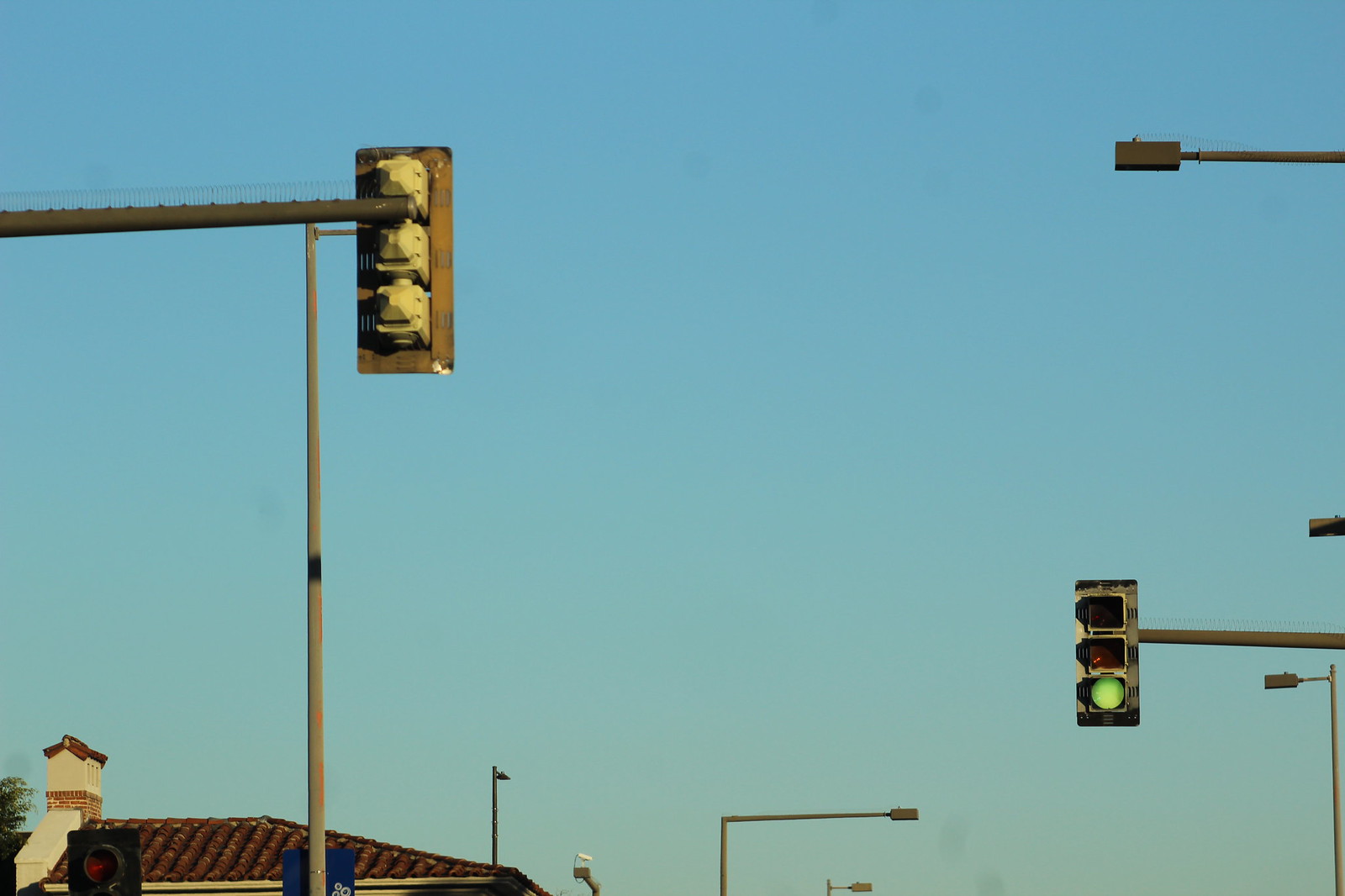This photograph captures a clear, cloudless daytime sky that transitions from medium blue at the top to a light blue-green hue nearer the bottom. Dominating the scene are traffic lights on horizontal poles, with notable fixtures visible throughout the image. 

In the top left corner, approximately 75% up the frame, there is the back side of a vertically mounted traffic light, extending horizontally into the shot. About a third of the way from the left, another traffic light is visible with the rear facing us, mounted on a horizontal pole.

In the lower right quadrant of the frame, positioned about a third up from the bottom and 25% in from the right, there is a traffic light facing towards the viewer, displaying an illuminated green light. Nearby and scattered throughout the background, multiple fixtures, potentially streetlights or sensors, are mounted horizontally, providing depth and context to the urban setting.

Additionally, in the lower left portion of the image, part of a Spanish missionary-style building with a terracotta tile roof and a small white chimney can be seen. Just above this building fragment, the top part of another traffic light is partially visible, with its red light illuminated. The meticulous details of the poles, lights, and structures provide a cohesive and intricate view of the city's traffic management system against the expansive clear sky.